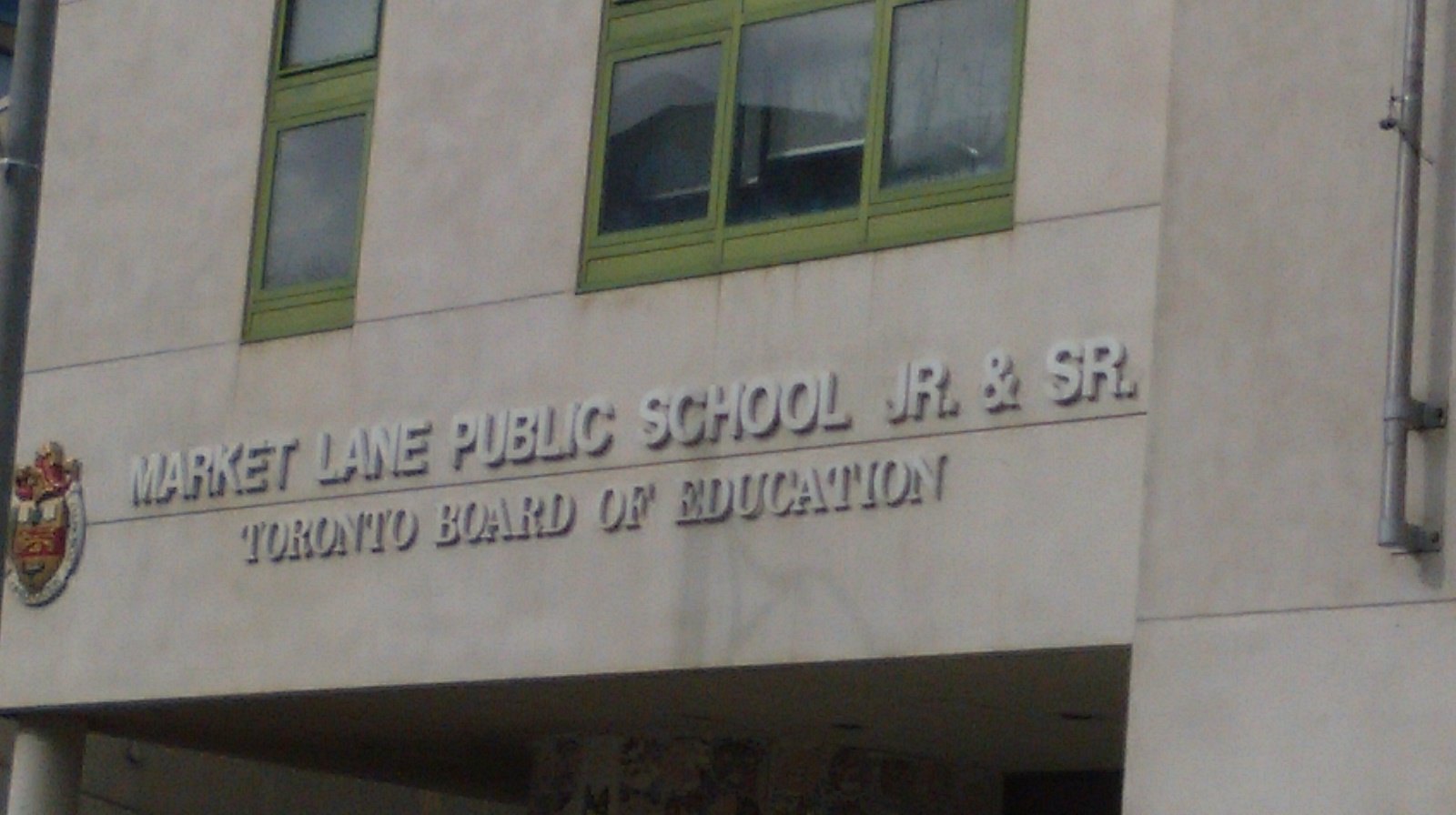This is a low-resolution, outdoor daytime photograph depicting the front facade of Market Lane Public School, Junior and Senior, part of the Toronto Board of Education. The building, made of grey concrete or painted in a greyish tone, features prominent green-trimmed window sets—one with three panes and another with two. Above the entrance, a sign clearly reads the school's name and its affiliation with the Toronto Board of Education. To the left of the text is a partially visible emblem adorned in red and gold, likely representing the city or district, though the details are unclear. To the right of the entrance, a flagpole is affixed to the building's wall, adding to the structural elements captured in this slightly angled photograph. The photograph does not feature any people, focusing solely on the architectural and identifying elements of the school building.